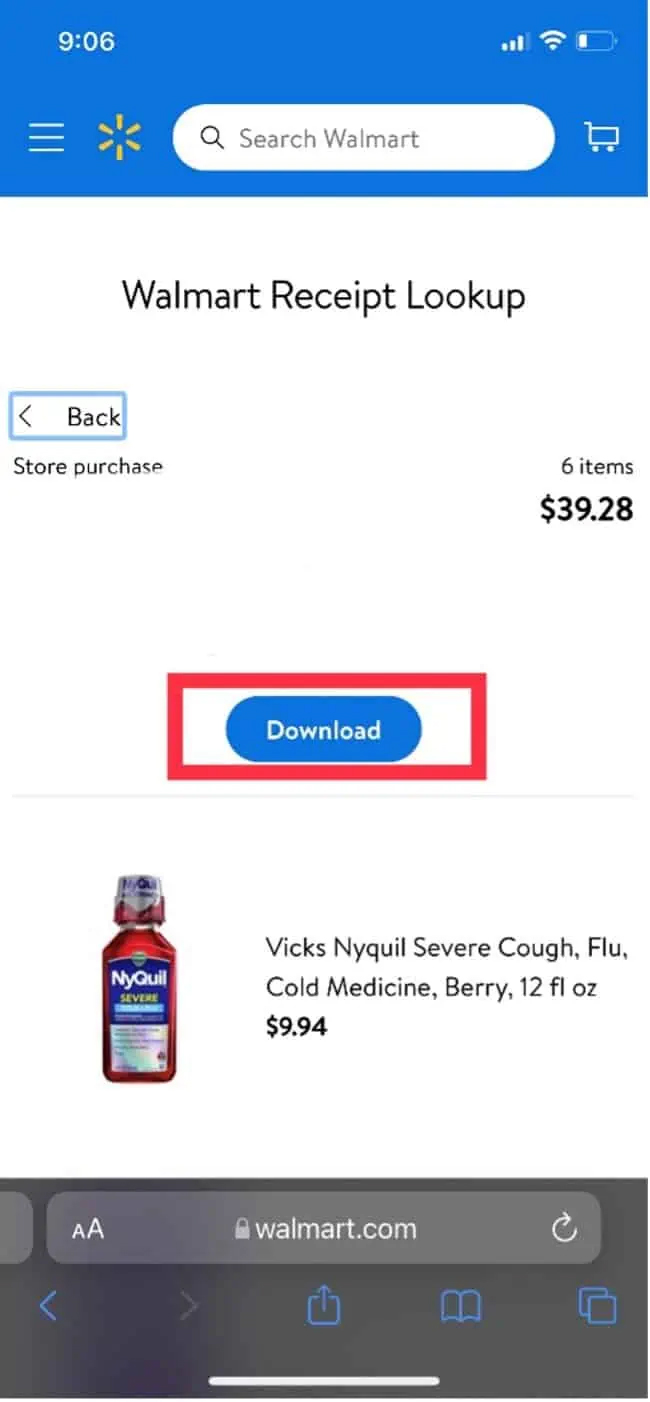This image depicts the receipt lookup page on the Walmart website, accessed via the Safari browser on a smartphone. The phone's status bar at the top has a blue background matching the Walmart search bar below it. The status bar displays a time of 9:06 AM, with a signal strength of 3 out of 4 bars, full Wi-Fi reception, and a battery level around 20%.

Below the status bar, the user interface includes a hamburger menu icon (three horizontal lines), the Walmart logo (a yellow burst of six lines), a capsule-shaped search bar, and a white shopping cart icon. The main heading reads "Walmart Receipt Lookup," and a blue-highlighted back button is visible to the left. The page details a recent purchase consisting of six items totaling $39.28.

A prominent blue capsule-shaped download button with white font is highlighted with a red rectangle. Below, a product listing features Vicks NyQuil Severe Cough and Flu Medicine in a 12 fluid ounce bottle. The liquid is red and the label is blue with "NyQuil" in white and "Severe" in yellow. The product description, "Vicks NyQuil Severe Cough Flu Cold Medicine Berry 12 fluid ounces," is in bold black font, priced at $9.94.

At the bottom, a gray rounded rectangle search bar reads "Walmart.com" accompanied by a padlock icon, indicating a secure connection. Additional icons for page refresh, sharing options, reading mode, and copy-paste features are present.